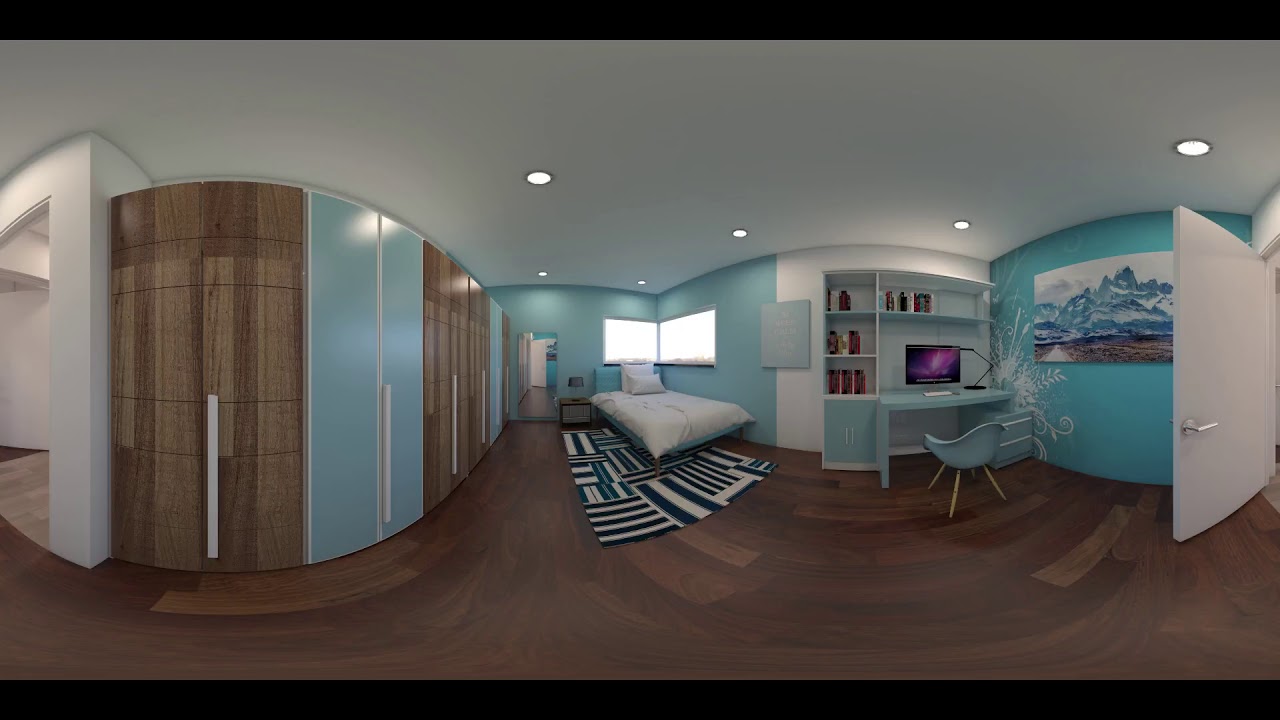The image showcases a uniquely distorted view of a room captured through a fisheye lens, emphasizing a sense of depth and curvature that warps the normal geometry. The room features alternating wooden and light teal wall panels, with the back wall being primarily teal. Two bright windows on the back wall illuminate a centrally placed bed adorned with white sheets and pillows. Directly beneath the bed is a patterned carpet with intersecting black, white, and teal lines, resembling a puzzle.

To the right, a blue chair sits in front of a blue desk, upon which a computer with a purple screen is situated. Above the desk, shelves display a collection of bottles, arranged in a staggered configuration. Further to the right hangs a painting of a snowy mountain landscape, adjacent to a white door with a silver handle.

The ceiling is white, with small circular lights casting a grayish shadow, and the floor boasts a wood grain finish. On the left side of the room, additional closet space and decorative shelving can be seen, with the shelving carrying more sculptures or similar objects. The combination of wall colors, furniture arrangement, and decorative elements contributes to a vibrant yet cozy atmosphere.